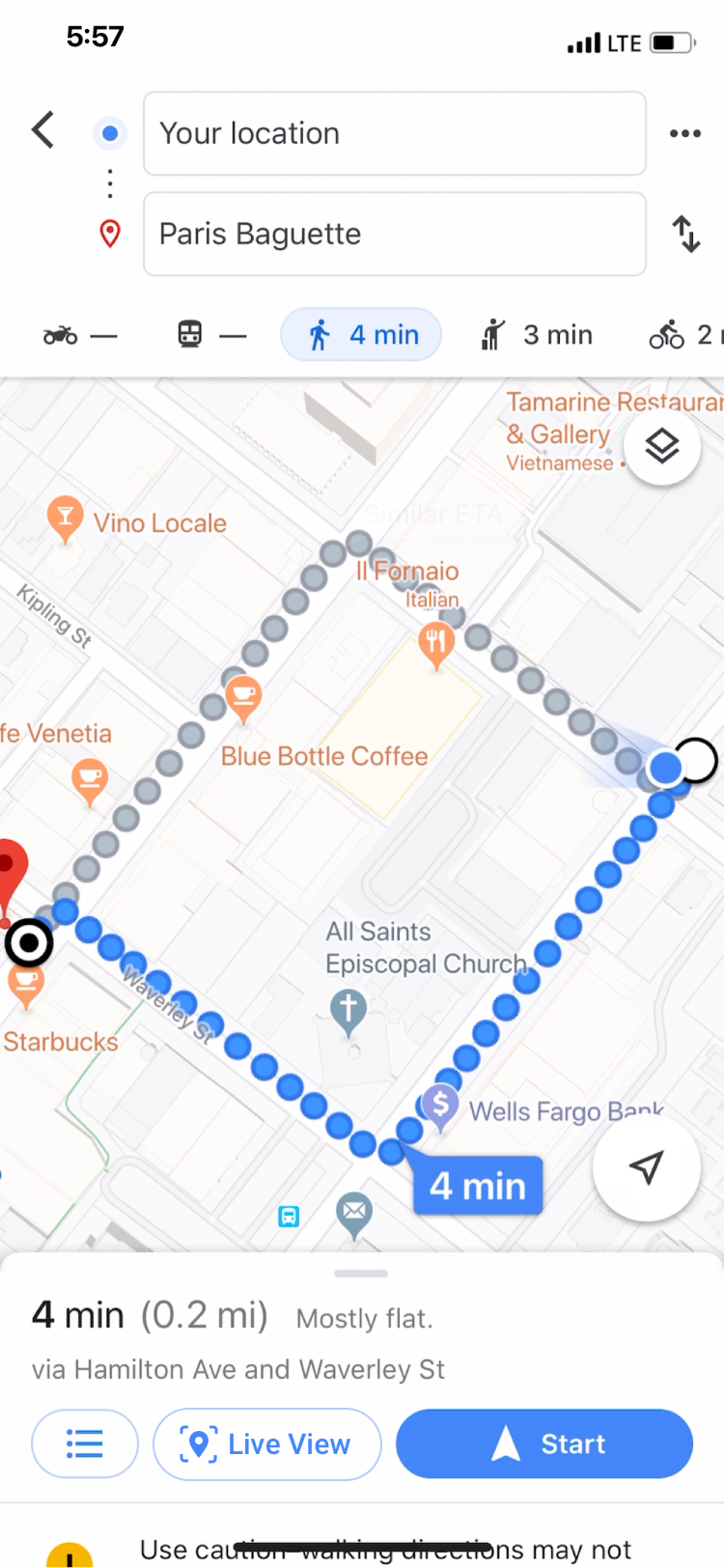A detailed depiction of a navigation screen on a digital device, possibly a tablet or smartphone, illustrating a walking route to Paris Baguette. 

In the upper left corner of the screen, the time is displayed as 5:57. The upper right corner shows essential status icons including cellular service bars, an LTE signal indicator, and a battery level at approximately 50%. Directly beneath these indicators, location data is shown with 'Paris Baguette' specified in the data field.

Below the location data, a row of transportation mode icons is present, portraying options for car, bus, walking, taxi, and bicycle. The walking icon is selected, prompting the display of walking directions. The route is visually represented on a map with a series of connected blue dots, outlining the path.

The walking route details state that it will take 4 minutes to cover a distance of 0.2 miles, predominantly along Hamilton Avenue and Waverly Street, which is mostly flat. Below the map and route details, there are additional options, formatted as bullet points for directions and a 'Live View' feature. 

A prominent blue button labeled 'Start' with white text and a white arrow invites the user to commence navigation. The color scheme of the display incorporates black, white, gray, blue, orange, yellow, and green. Lastly, a cautionary note advises users to exercise caution.